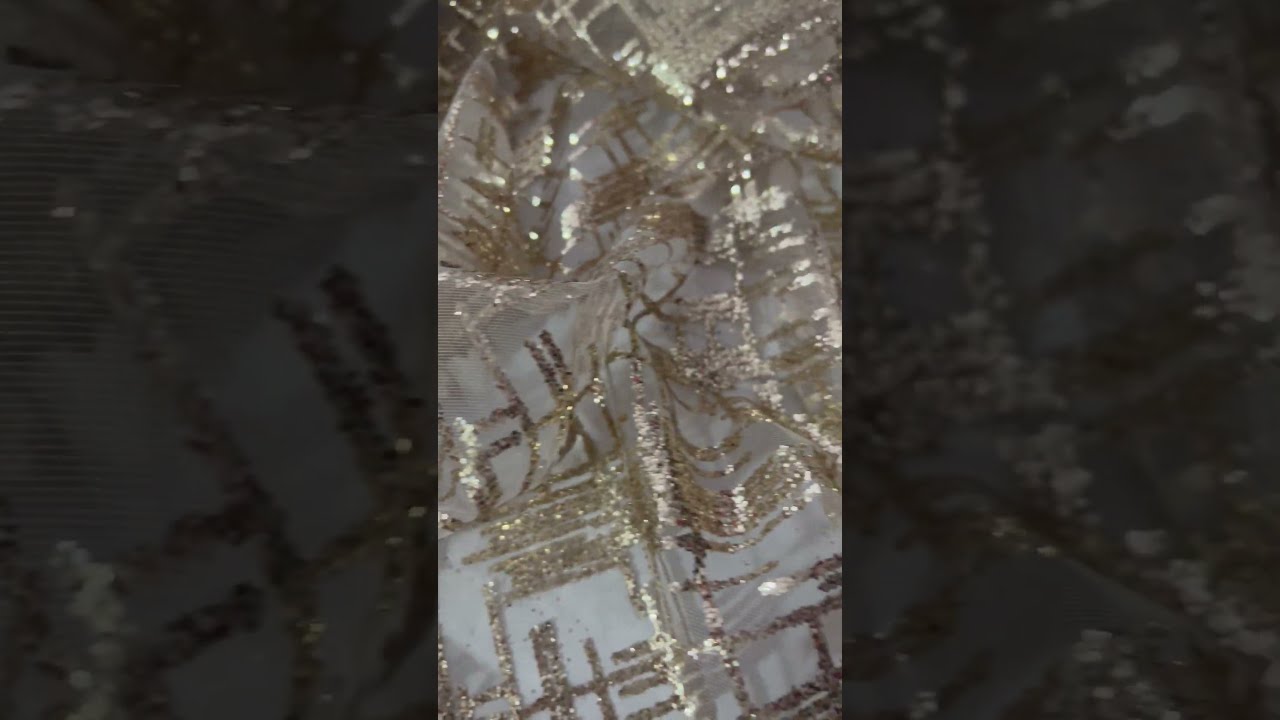This rectangular image is divided into three vertical sections, where the outer left and right sections feature darkened close-ups of the central image. The centerpiece is a crinkled and folded piece of transparent, white net-like fabric adorned with a glittery, metallic gold design. The design appears geometric, with lines, squares, 90-degree angles, and parallel lines, and might resemble a decorated ribbon at the top. The fabric has a shiny, textured look, evoking a festive holiday theme, such as Christmas or New Year's. The entire image focuses solely on this glittery, gold-and-white patterned fabric, with no background distractions.